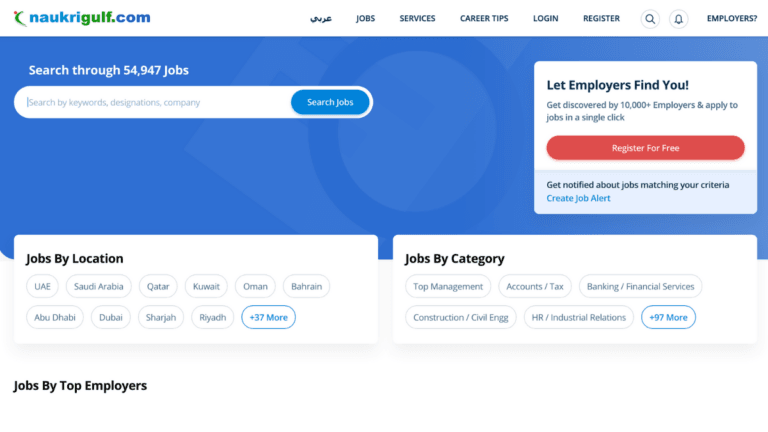This image features a screenshot of the website naukrigulf.com, a job portal targeting the Gulf region. At the top of the page, there is a navigation bar with clickable options, including "Categories," "Jobs," "Services," "Career Tips," "Login," "Register," a search icon, a notification bell, and "Employers?" with a question mark.

Below this navigation bar, on a blue background, there is a prominent search area inviting users to "Search through 54,947,000 jobs." This search functionality allows users to type in their queries and then click the "Search Jobs" button.

Adjacent to the search area, on the right side of the blue box, is a white informational box featuring text in black and gray. The text encourages users to: "Let employers find you, get discovered by 10,000+ employers, and apply to jobs in a single click." It also highlights the option to "Register for free" in red text. Additionally, it mentions that users can get notified about jobs matching their criteria and create job alerts.

Below this section, there are two rectangular clickable areas. The first one, "Jobs by Location," lists various countries, allowing users to find job opportunities by geographical area. The second one, "Jobs by Categories," categorizes job types such as "Top Management," "Accounts/Tax," "Banking," and "Financial Services," among others. Both sections provide more options within each category for users to explore further.